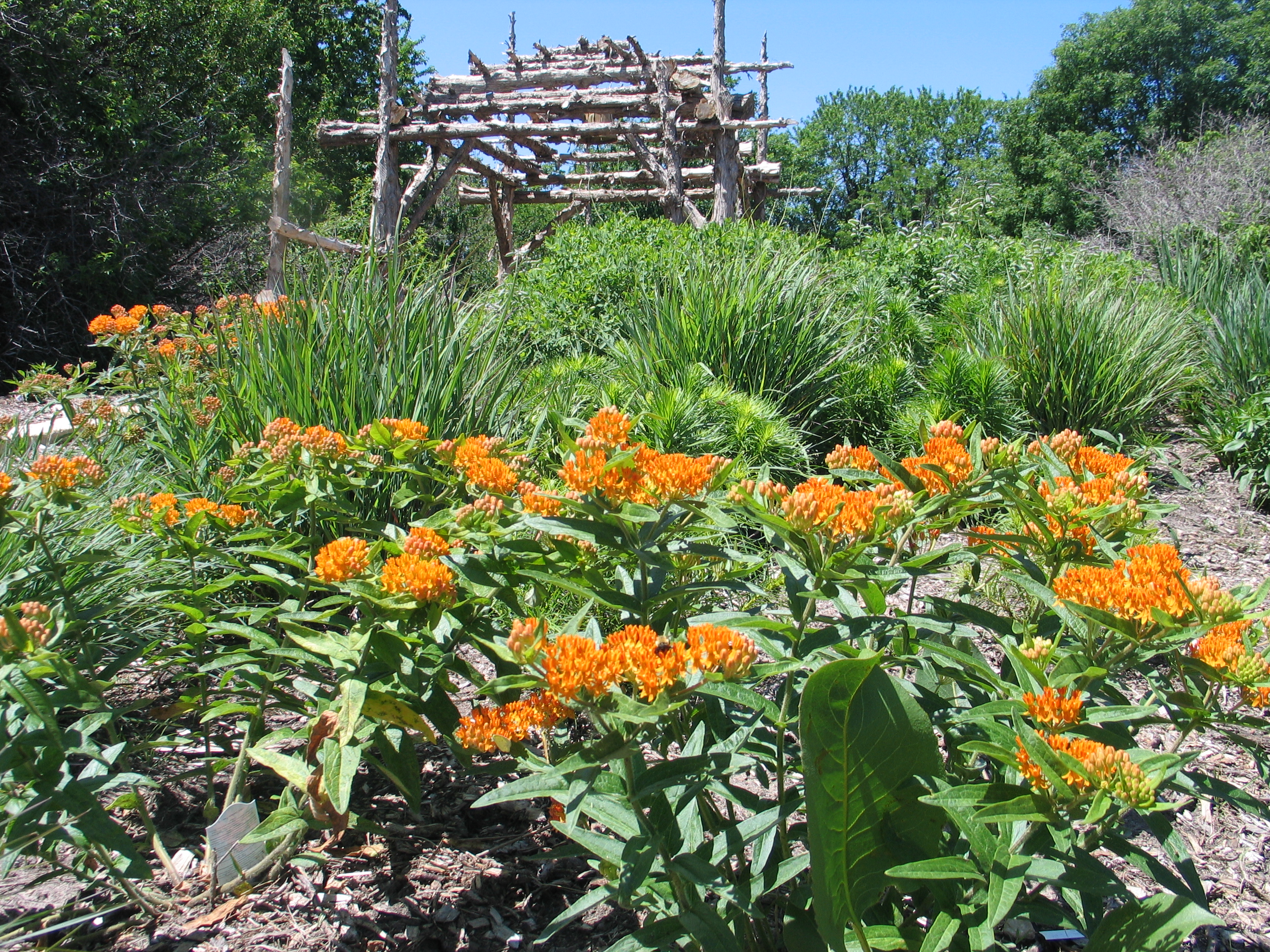The image depicts a vibrant outdoor scene bathed in midday sunlight with a clear, blue sky. In the foreground, there is a prominent cluster of blooming orange flowers, complete with varying shades of yellow at their tips and surrounded by large, lush green leaves. These flowers are scattered amongst wood chips and some dried grass or leaves. Nearby, an intriguing yet dilapidated wooden framework, resembling a small stick house with no doors or clear purpose, stands amidst the lively environment. Surrounding the structure are numerous knee-high green plants and dense bushes, all teeming with life. In the background, a variety of green trees provide a rich, verdant backdrop to this serene, nature-filled scene.